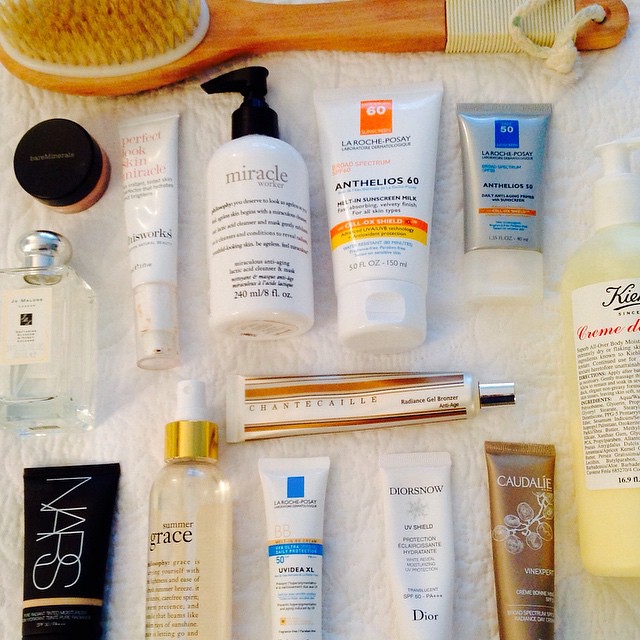This top-down photograph showcases a white towel meticulously spread out, adorned with an assortment of tubes and bottles, predominantly cosmetic products. At the very top of the composition, there's a wooden-handled brush wrapped in a fabric tape near its top, with bristles in a striking orange-brown hue.

In the array of cosmetics, several products stand out. Among them are:

1. A tube labeled "Perfect Look Skin Miracle".
2. A white bottle prominently featuring "Miracle Worker, 240mg, 8 fluid ounces".
3. An orange-capped tube with the number "60" inscribed on it.
4. Multiple products from La Roche-Posay, including:
   - A bottle with the text "La Roche-Posay Laboratoire Dermatologique", "Anthelios 60", and "Melt-In Sunscreen Milk", detailing its content as "5 fluid ounces".
   - A smaller tube to the right bearing "50" in blue, part of the Anthelios line.

Additionally, there are several other colorful tubes and bottles scattered meticulously across the towel, creating an organized yet visually captivating collection of cosmetic essentials. The overall scene exudes a sense of indulgence in skincare and beauty routines, highlighted by the neat presentation and diversity of products.